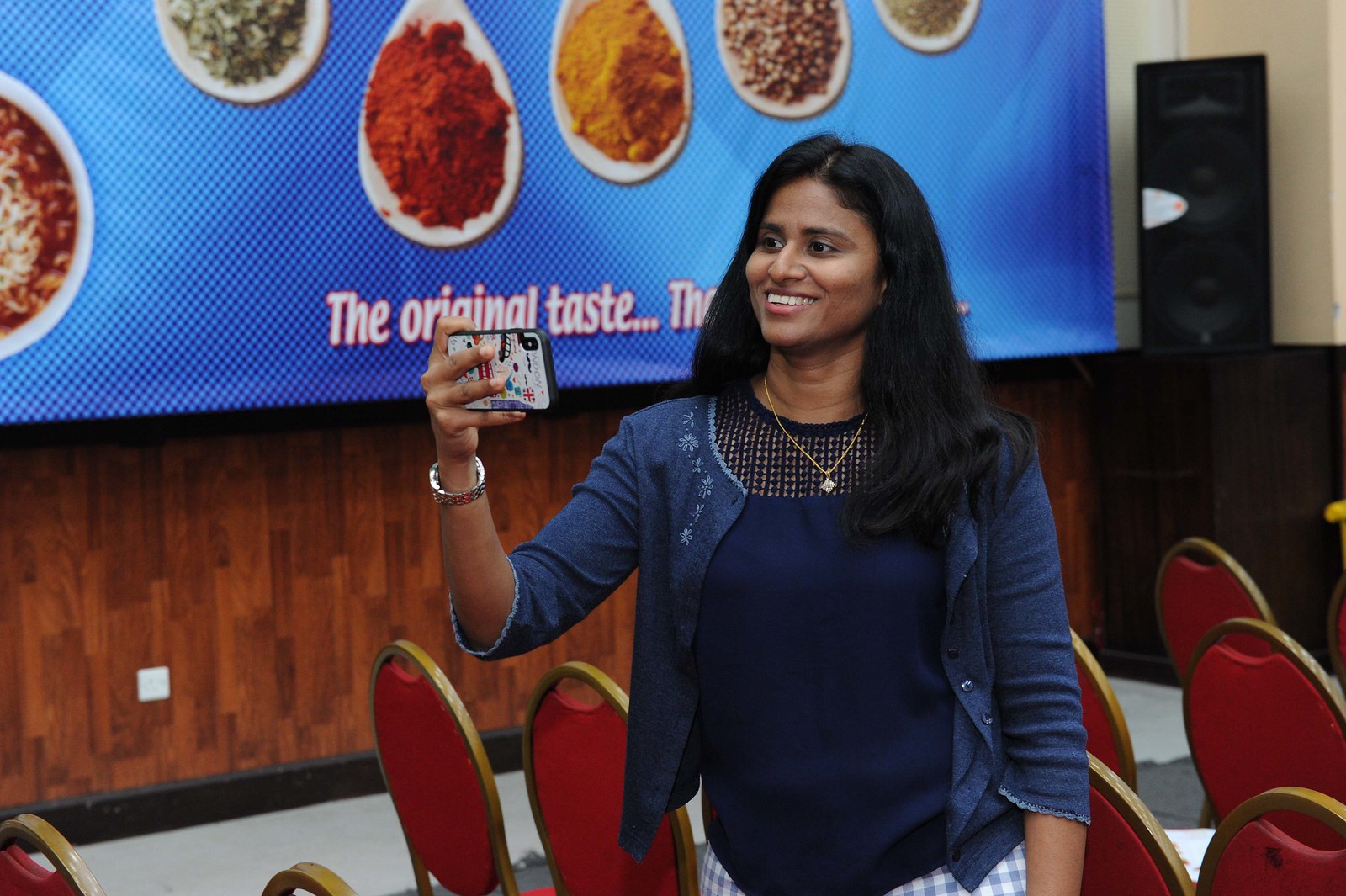In the photo, a brown-skinned woman with long, dark black hair stands indoors, smiling at her cell phone as she takes a selfie. She is wearing a blue top with a netted upper section beneath a button-down blue jacket with 3/4 sleeves. A watch adorns her right wrist, and she is accessorized with a necklace. She appears to be in a conference room or similar setting, characterized by multiple red, oval-shaped chairs with gold trim arranged around her. The space has wood paneling on the walls and a gray floor with black baseboards. Behind her, a large blue banner depicts various spices and possibly food items, with text that reads "The Original Taste..." partially obscured by her head.